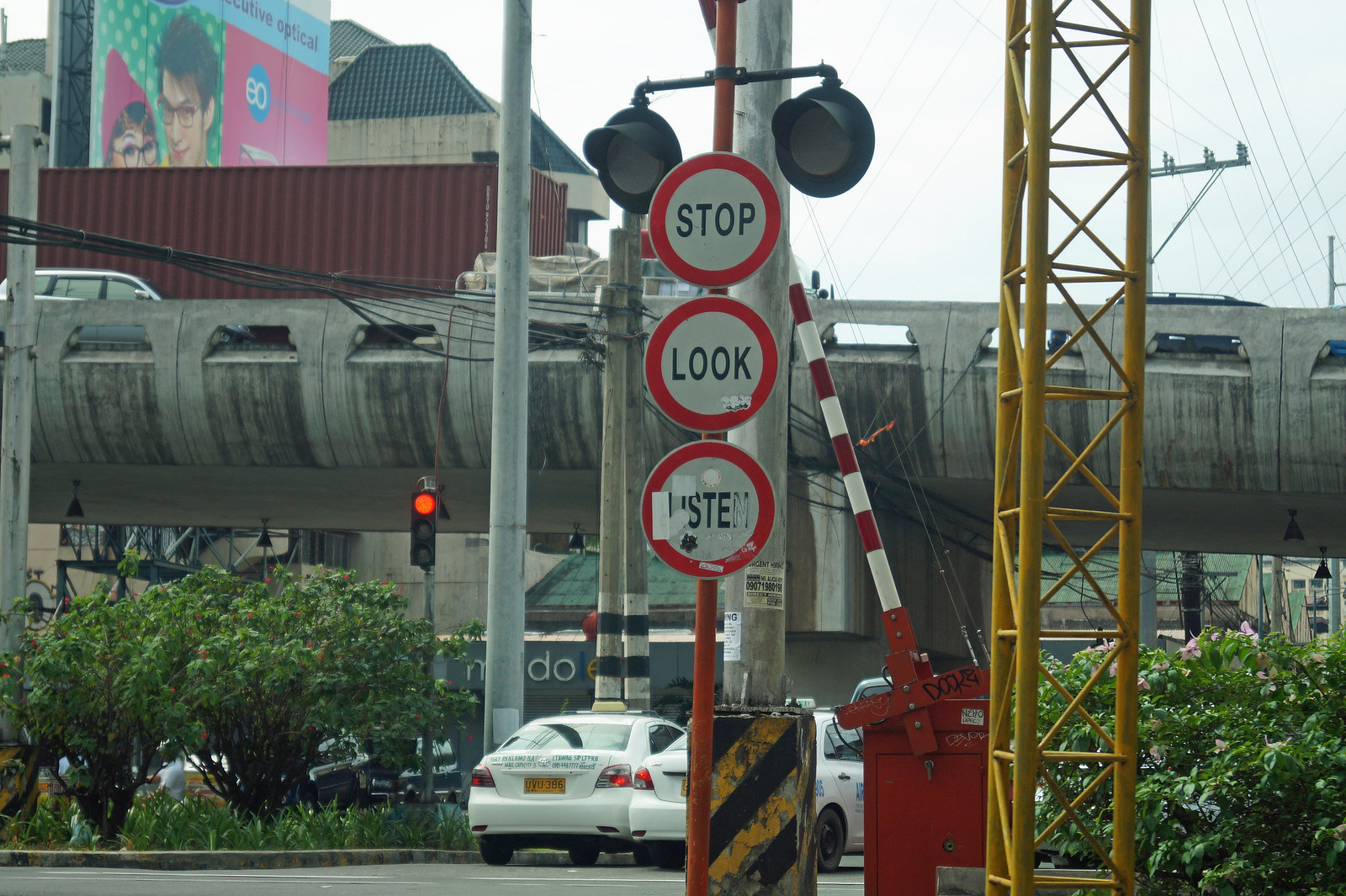The image depicts a bustling, industrial town featuring a central concrete bridge that spans horizontally across the middle of the scene. Below the bridge, a small traffic jam is evident as cars halt at a red traffic light. The bridge is a focal point, complemented by a large red-and-white barrier arm to the right, designed to prevent vehicles from crossing during train passages. Prominent in the foreground is a distinct vertical pole adorned with three circular signs that sequentially read "Stop," "Look," and "Listen," emphasizing railway safety.

Further back, visible through the urban clutter, a reddish-brown shipping container adds an industrial touch, though it is unclear what platform it rests on. Vegetation, including small trees, frames the scene on the left and right, lending a touch of greenery to the urban landscape.

Above it all, a clear white sky forms the backdrop for a large billboard advertising optical products, located in the upper left-hand corner. The advertisement features the faces of a Caucasian man and woman, both sporting glasses, capturing attention with an implied message about eyewear. Additionally, the billboard appears to contain Japanese characters, suggesting perhaps an advertisement in a multicultural area. This detailed and layered scene merges industrial elements with everyday urban life, underpinned by a sense of organized chaos.